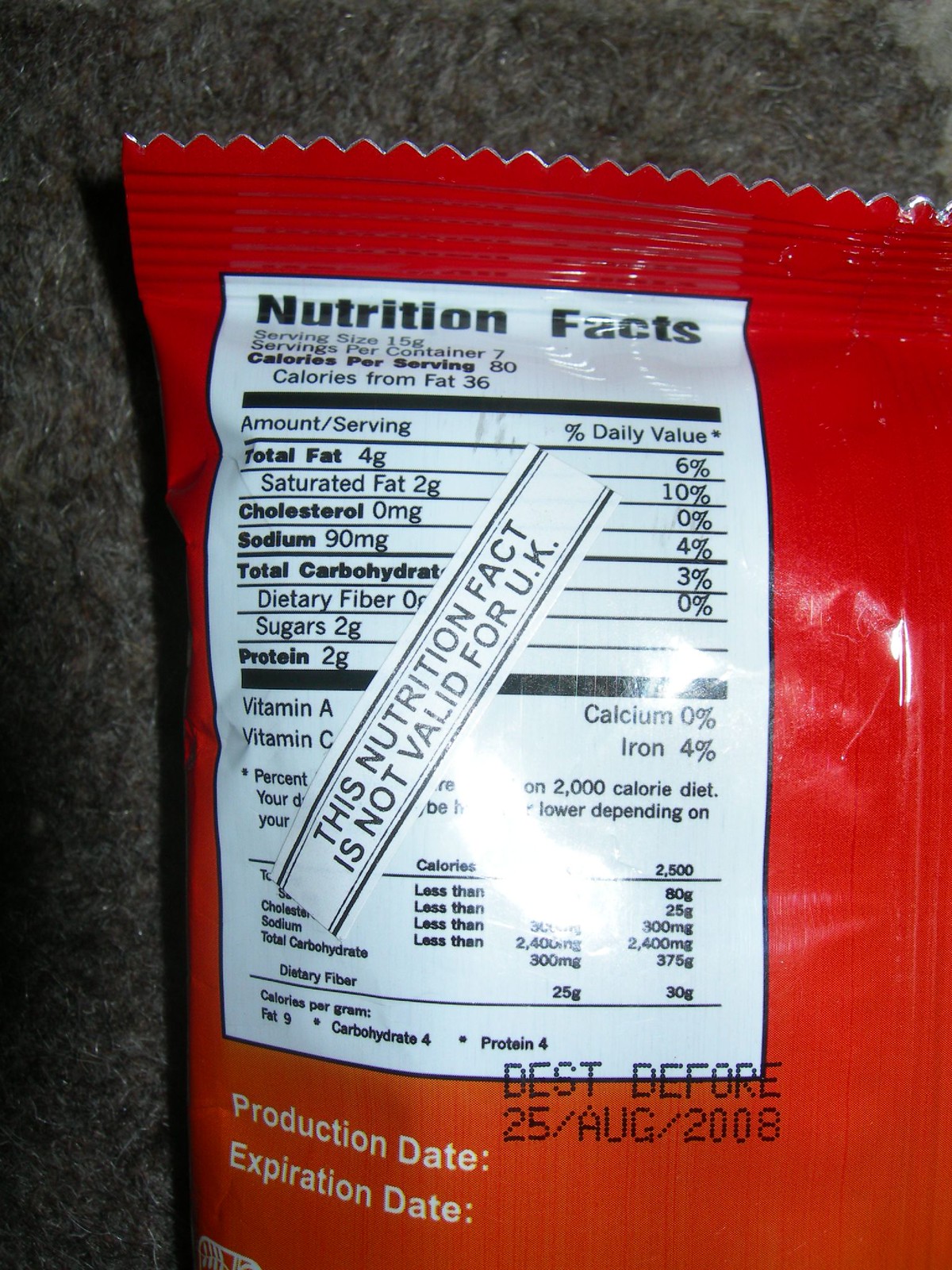The image depicts a red package, the exact content of which is unidentified. Prominently displayed are the nutritional facts, formatted in the standard black and white layout familiar in the United States. However, this information is partially obscured by a vertically placed sticker, reminiscent of a U.S. Surgeon General warning. The sticker explicitly states that the listed nutritional information is not valid in the U.K., highlighting the United Kingdom's stricter nutritional regulations compared to those in the United States. In the bottom right corner of the package, a stamp indicates "Best before 25 August 2008," overlapping with the nutritional label. There are also designated spaces for the production and expiration dates, but these details are cropped out of the image, rendering them illegible.